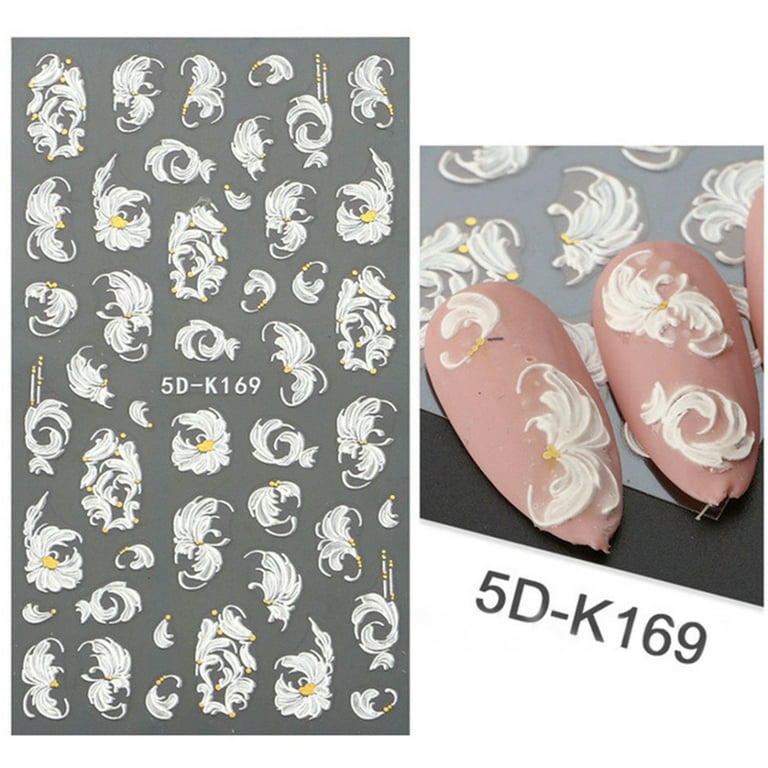This image appears to be an advertisement or promotional display for a nail salon, showcasing various floral nail design options. On the left side, there is a large gray panel featuring rows of intricate, white floral designs with a yellow dot in the center of each flower. These designs vary in shape and size but all share a delicate, petal-like motif. On the right side, these floral designs are displayed in close-up on what seem to be artificial nails, finished with a soft pink base. These nails are positioned on a dark black table, and beneath them is a code, 5D-K169, which matches the code displayed on the large gray panel. This display likely serves as a catalog for potential customers to select their desired nail designs at the salon.